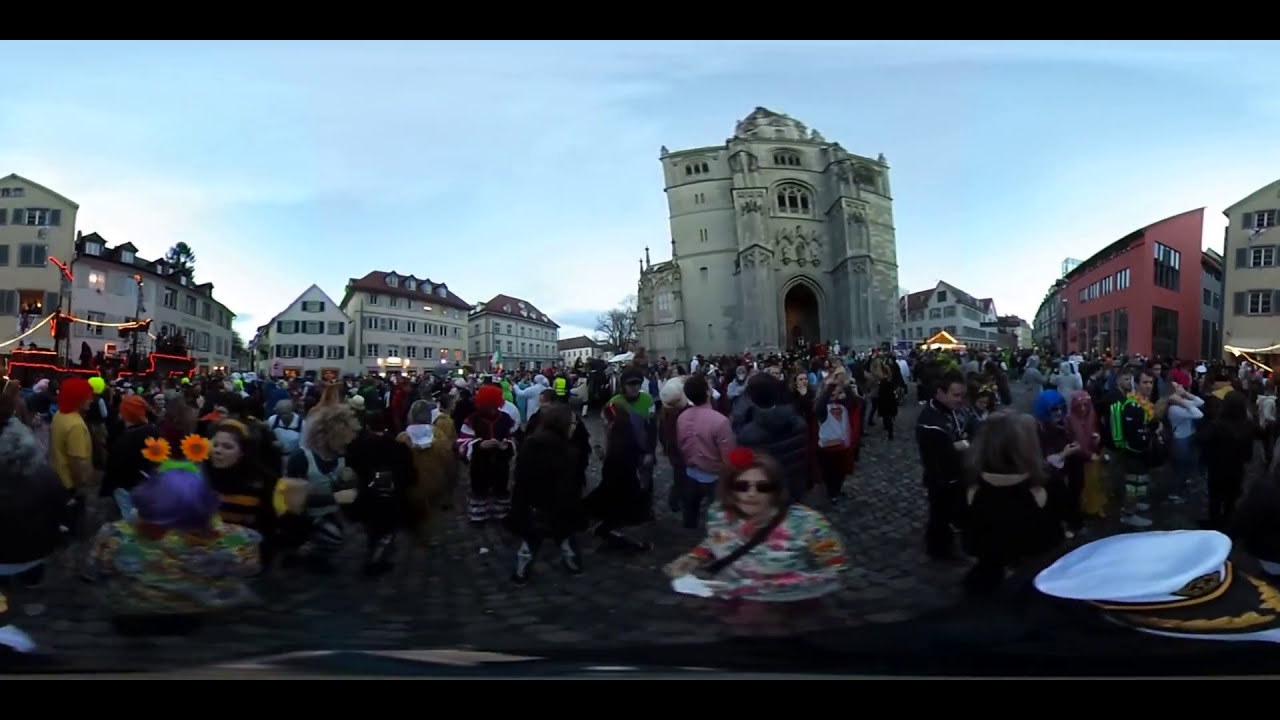This wide rectangular panoramic photograph captures a vibrant scene in a European town square, likely during a festive event. The bottom half of the image showcases a bustling crowd of people, many dressed in colorful costumes and fun outfits, standing on a cobblestone road that exhibits some distortion, possibly due to the use of a 360-degree or 180-degree camera. Prominently visible in the bottom right corner is a white military or naval cap with black and gold trim. Central to the scene is a woman in a green, pink, and white floral print shirt, adorned with a red carnation in her hair and wearing sunglasses, with a bag slung over her right shoulder.

In the distance, a large, ornate stone building with a towering archway, likely a church, anchors the composition slightly to the right of center. On the left side of the image, several multi-story white buildings with red roofs line the square, while a colorful strip of lights outlines a pirate ship, possibly a float, hinting at a celebration or festival. Towards the right, additional multi-story buildings in hues of red, yellow, and brown line the street. The sky overhead is a bright blue, transitioning to lighter shades closer to the rooftops, underscoring the daytime setting.